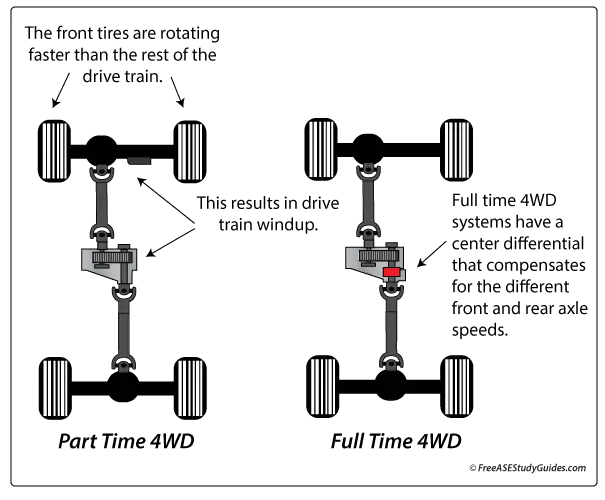The diagram provides a detailed comparison between part-time and full-time four-wheel drive systems, highlighting the undercarriage and mechanical workings of each. The left side of the diagram, labeled "part-time 4WD," illustrates the front tires rotating faster than the rest of the drivetrain, leading to drivetrain windup. Arrows and accompanying text highlight key components and issues. The right side, labeled "full-time 4WD," shows a similar undercarriage but includes a center differential, colored in red, which compensates for different front and rear axle speeds. The text clearly explains the functionality of the center differential in managing axle speed discrepancies. The diagram is set against a white background, bordered in black, with annotations and arrows in black for clarity. Additionally, small text in the bottom right corner credits ASE StudyGuides.com.